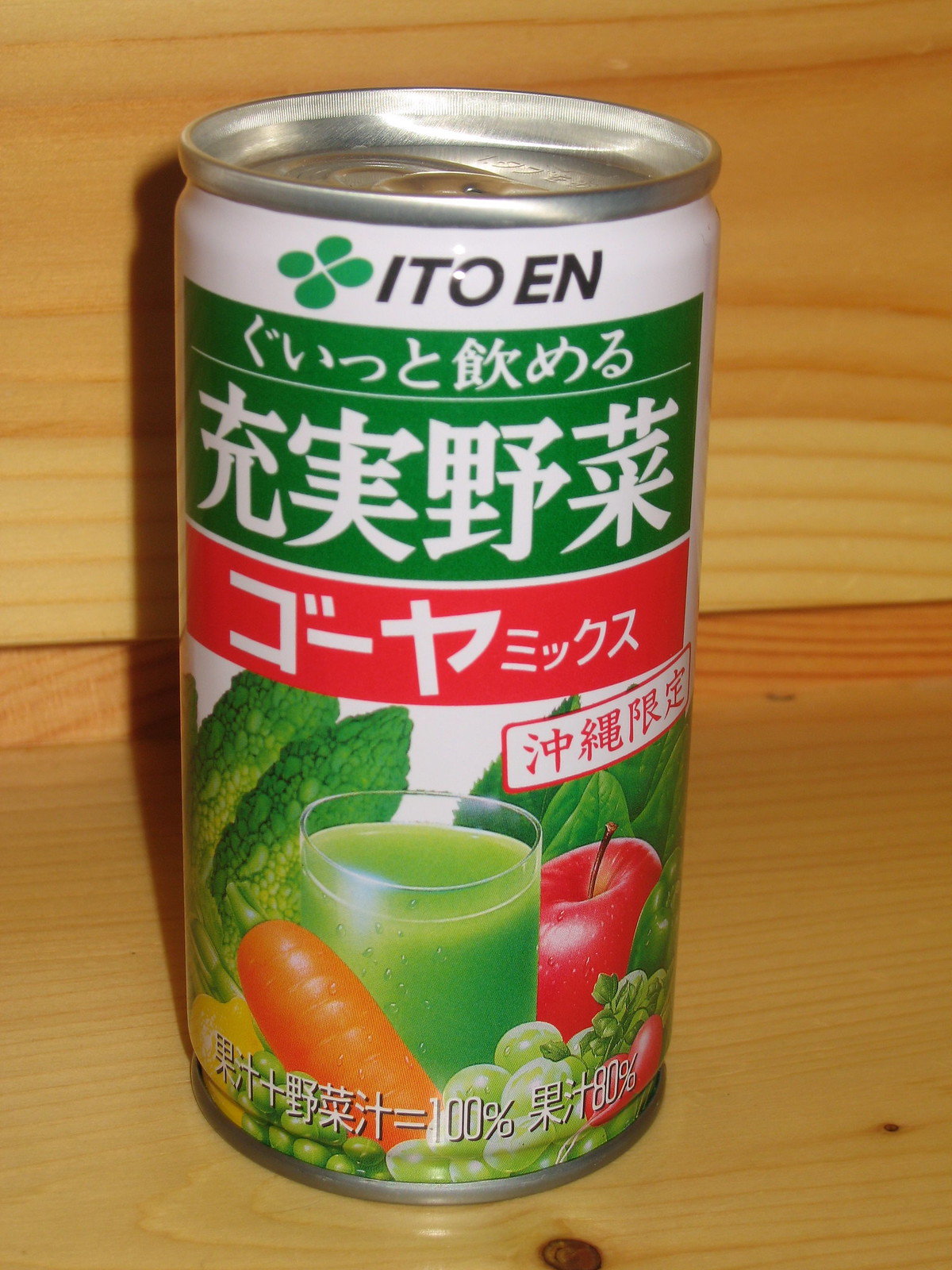A photograph captures an intricately detailed, vibrant beverage can of probable Asian origin, adorned predominantly with Mandarin script. The sleek, pop-top can, which appears to hold approximately 16 ounces, features a striking green and white color scheme—green elements richly interspersed with white background areas. A red label further accentuates the can, housing a portion of the text. Predominantly green-themed, the can showcases a stylized image of a glass filled with a green liquid, hinting at the beverage's contents. Surrounding this image are illustrations of various fresh produce including grapes, carrots, leafy greens, an apple, and a tomato. The bottom portion of the can reveals numerical information, potentially percentages, rendered in an eye-catching layout. The overall design is dynamic and engaging, projecting a sense of natural, wholesome vitality.